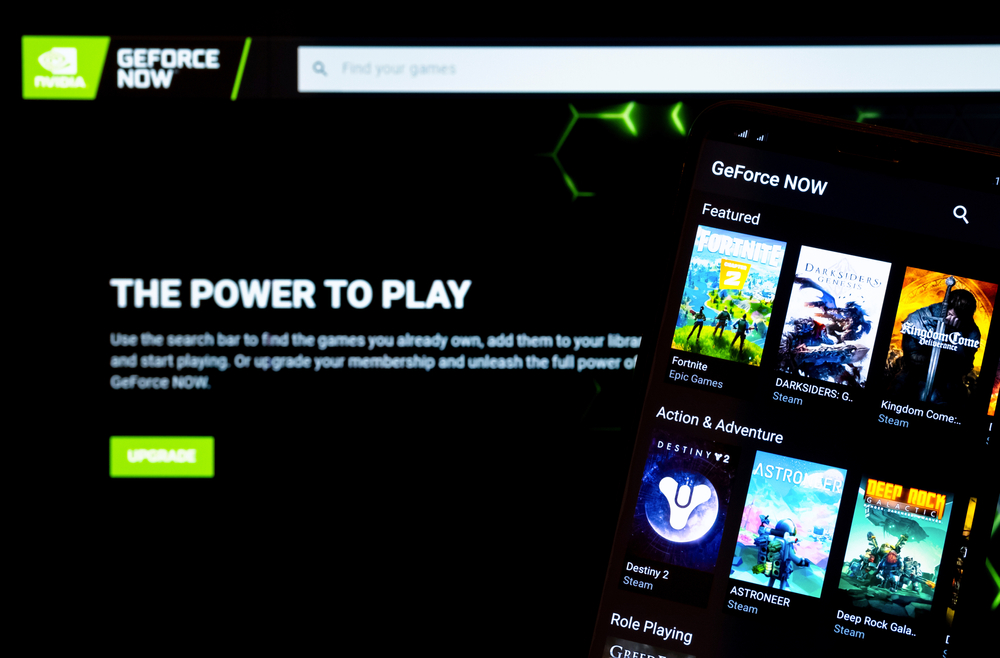A detailed caption for the image could be:

"This is a widescreen color screenshot of a website. At the top of the page, the text 'GEFORCE NOW' is prominently displayed in white against a dark background, accompanied by a neon green diagonal slash that adds a dynamic element to the header. Directly below this, a search bar is available with the placeholder text 'Find your games' to guide users. 

The website's central message, also in white, reads 'The power to play.', followed by instructions: 'Use the search bar to find the games you already own, add them to your library, and start playing. Or upgrade your membership and unleash the full power of GEFORCE NOW.' Below this text, a green banner with white text urges users to 'Upgrade' their membership.

To the right of the text, a collage of various game covers is displayed, showcasing featured games available on the platform. The featured games include 'Fortnite' (from Epic Games), 'Darksiders' (on Steam), 'Kingdom Come Deliverance' (on Steam), 'Destiny 2' (on Steam), 'Astroneer' (spelled out as A-S-T-R-O-N-E-E-R, on Steam), and 'Deep Rock Galactic' (also on Steam). These game covers are accompanied by corresponding platform labels and genre tags such as 'Action and Adventure.'

At the bottom of the image, partially cut-off text hints at more information about role-playing games and additional content not fully visible in the screenshot. The image contains no animals, plants, flowers, trees, buildings, or motorized vehicles, emphasizing its focus on digital content.